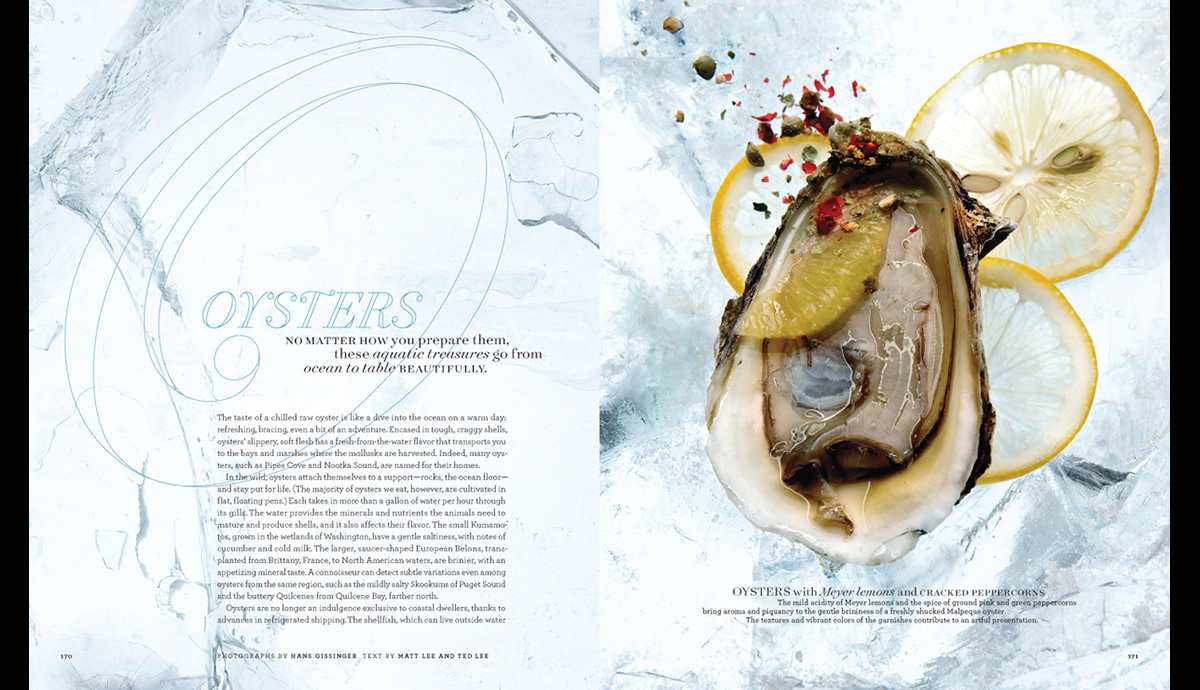The web page is designed with a unique aesthetic, resembling a book rather than a traditional website. On the left side of the page, a section aptly titled "Oysters" features an evocative description: "No matter how you prepare them, these aquatic treasures go from ocean to table beautifully." Adjacent, on the right side, is a stunning photograph showcasing a freshly shucked oyster, complemented by three thinly sliced lemon wedges and a sprinkling of powdered chilies.

Below this image, the left side text continues to captivate the reader, describing the sensory experience of indulging in a chilled raw oyster: "The taste of a chilled raw oyster is like a dive into the ocean on a warm day—refreshing, exhilarating, even a bit of an adventure." It poetically illustrates the oysters' journey from their tough, craggly shells to the table, emphasizing their fresh-from-the-water flavor that mentally transports diners to the bays and marshes where these mollusks are harvested.

The narrative adds depth by mentioning various oysters like Pipes Cove and Notok Sound, which are named after their habitats. It explains that while wild oysters attach themselves to rocks or the ocean floor for life, the majority consumed today are cultivated in flat, floating pens. Impressively, each oyster processes over a gallon of water per hour through its gills, extracting minerals and nutrients from the ocean-filtered water.